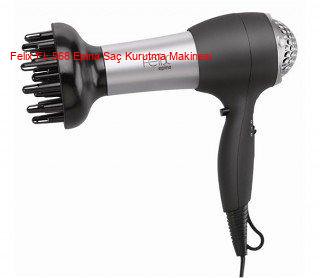The image shows a detailed product photograph of a hairdryer, captured at an angle that reveals its black handle and shiny silver body. The rear screen covering the intake, also silver, features rounded vent holes. The main barrel of the hairdryer has a sleek, satin finish and is equipped with a black, cup-shaped diffuser featuring several long plastic fingers extending from it, designed to aid in styling. The black power cord extends from the handle's bottom and falls out of the frame. Overlaid in small, red font across the silver barrel is some text, which is not entirely legible but seems to include the brand name "Felix" and possible foreign words written in English letters.